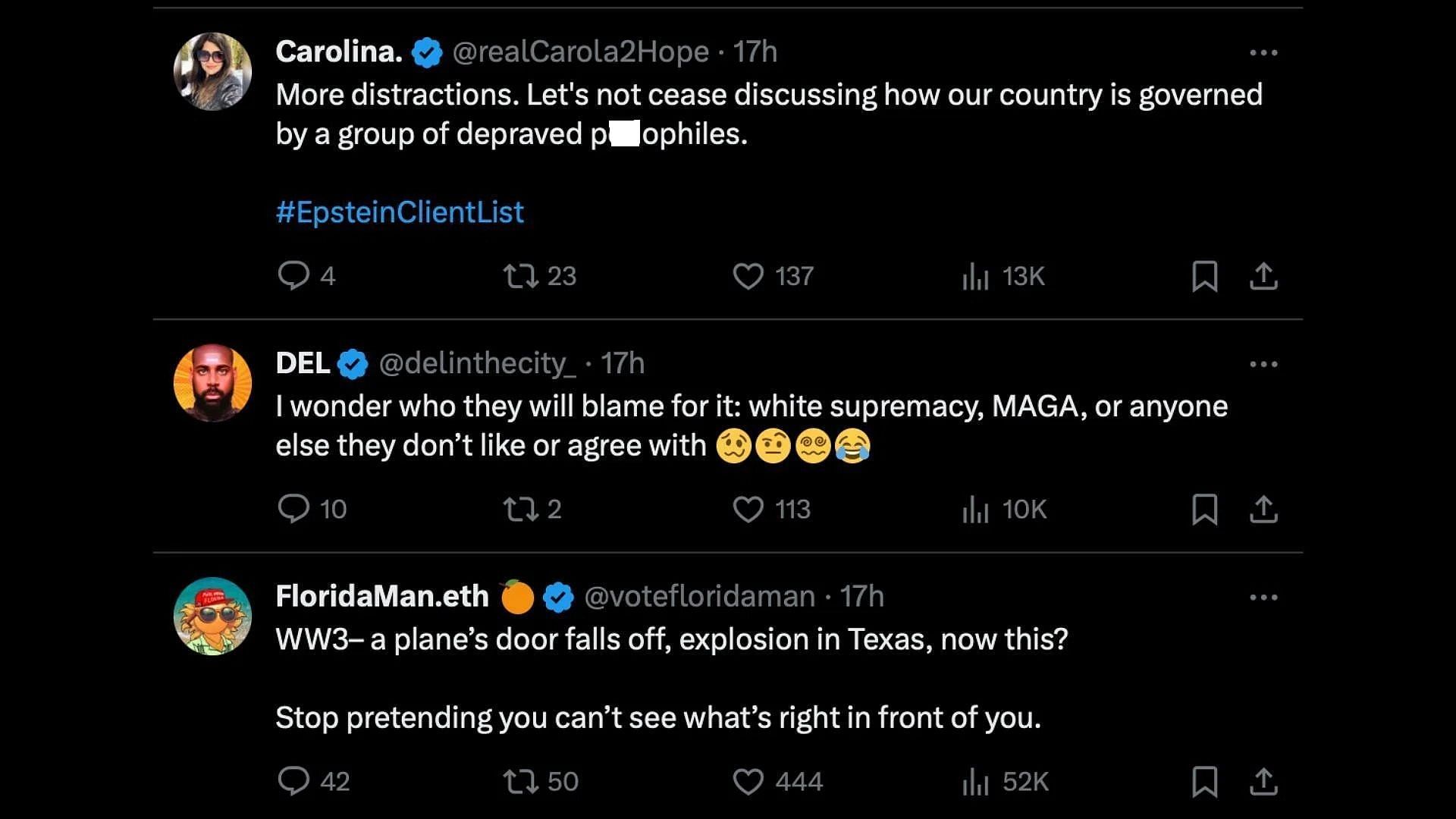**Photographic Image: Detailed Conversation Screenshot Description**

In this image, we see a captured screenshot of an online conversation against a black background. On the left side, there's a chat bubble containing a profile picture of a woman with dark hair and sunglasses. Her name is Carolina (or Carolina), and she is a verified user. Her handle reads "realCorollaToHope17."

Carolina’s message reads: "More distractions. Let's not cease discussing how our country is governed by a group of depraved pedophiles. #EpsteinClientList." The hashtag "#EpsteinClientList" is hyperlinked for further navigation.

Below her message, the engagement metrics are displayed: 4 comments, 23 shares, 137 likes, and 13,000 views. There are options available for bookmarking and sharing this post.

To the right of Carolina's message, another profile bubble shows a man with a full beard against a yellow background. He is an African-American man named Del, who is also a verified user. His handle is "DelInTheCity." Seventeen hours ago, Del responded with the following message: "I wonder who they will blame for it. White supremacy, MAGA, or anyone else that don't like or agree with." He included several emojis: a queasy face, an inquiry face, a dizzy face, and a laughing-crying face.